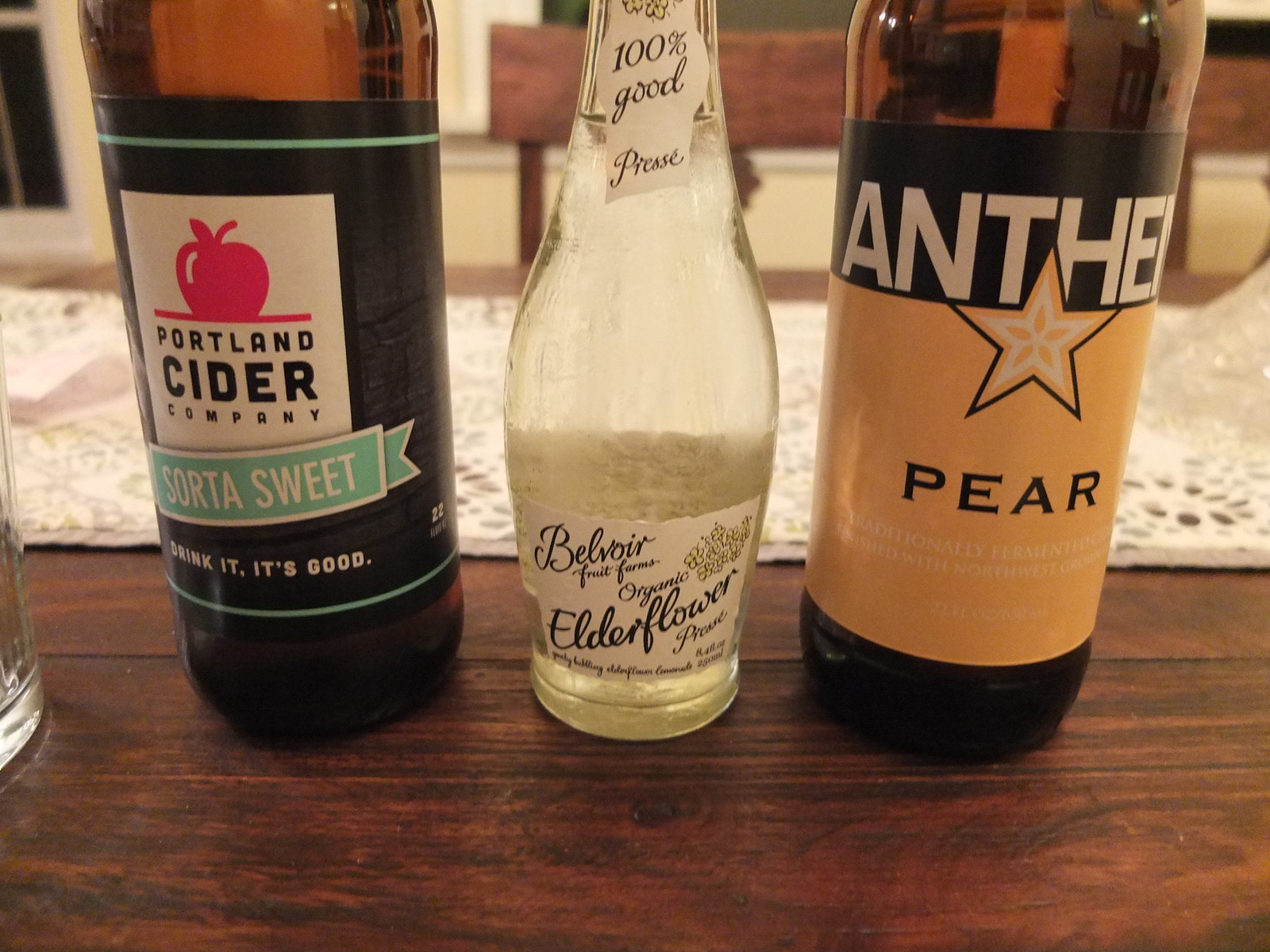This photograph displays three distinct bottles of alcoholic beverages arranged on a darker wooden dining table with a white table runner in the background. The first bottle on the left is from the Portland Cider Company, featuring a black label adorned with a red apple image and turquoise outlines. The label includes the phrases "Sorta Sweet" and "Drink It, It's Good" in white lettering, adding a touch of encouragement for the drinker. The bottle itself is copper-colored with a clear liquid inside.

In the center, there's a smaller, clear glass bottle that exudes elegance. It's labeled "Belvoir Fruit Farms Organic Elderflower." The label has a sophisticated, French-like design, and the liquid inside appears as a bubbly, yellowish-clear color, reminiscent of white wine or a sparkling beverage.

The third bottle on the right showcases a darker brown glass with a black label featuring an orange section and a star. It distinctly reads "Anthem Pear" and includes descriptions like "Traditionally Firm," although the full details are partially obscured due to the bottle's curvature. This bottle follows the copper color theme, housing what appears to be another clear liquid inside.